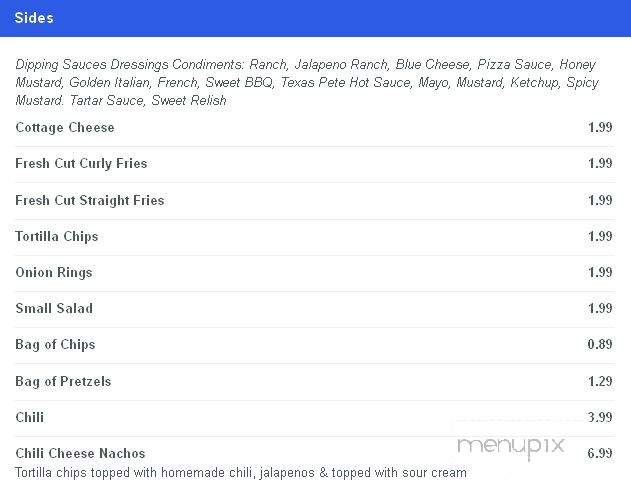### Detailed Caption for Image

This image is a screenshot of a segment from a menu, specifically focusing on the "Sides" category. The top part features a prominent blue box with the word "SIDES" displayed in white, aligned to the left. Directly below this, there is a section in italics listing various dipping sauces, dressings, and condiments including ranch, jalapeño ranch, blue cheese, pizza sauce, honey mustard, golden Italian, French, sweet barbecue, Texas Pete hot sauce, mayo, mustard, ketchup, spicy mustard, tartar sauce, and sweet relish. However, this italicized text appears somewhat blurry and difficult to read, indicative of a poor-quality screenshot.

Below the category header, there is a list of sides presented in a darker and bolder font. The text here is not perfectly clear either, as it appears light and slightly skewed, possibly due to printing errors. The listed sides include cottage cheese, French curly fries, fresh-cut curly fries, fresh-cut straight fries, tortilla chips, onion rings, small salad, bag of chips, bag of pretzels, chili, and chili cheese nachos. Prices for these items are aligned vertically along the right-hand side of the list.

The image also includes a watermark in the bottom right corner that reads "MENU PIX" in light gray, suggesting the source might be a website. Each menu item is separated by a light gray line for clarity.